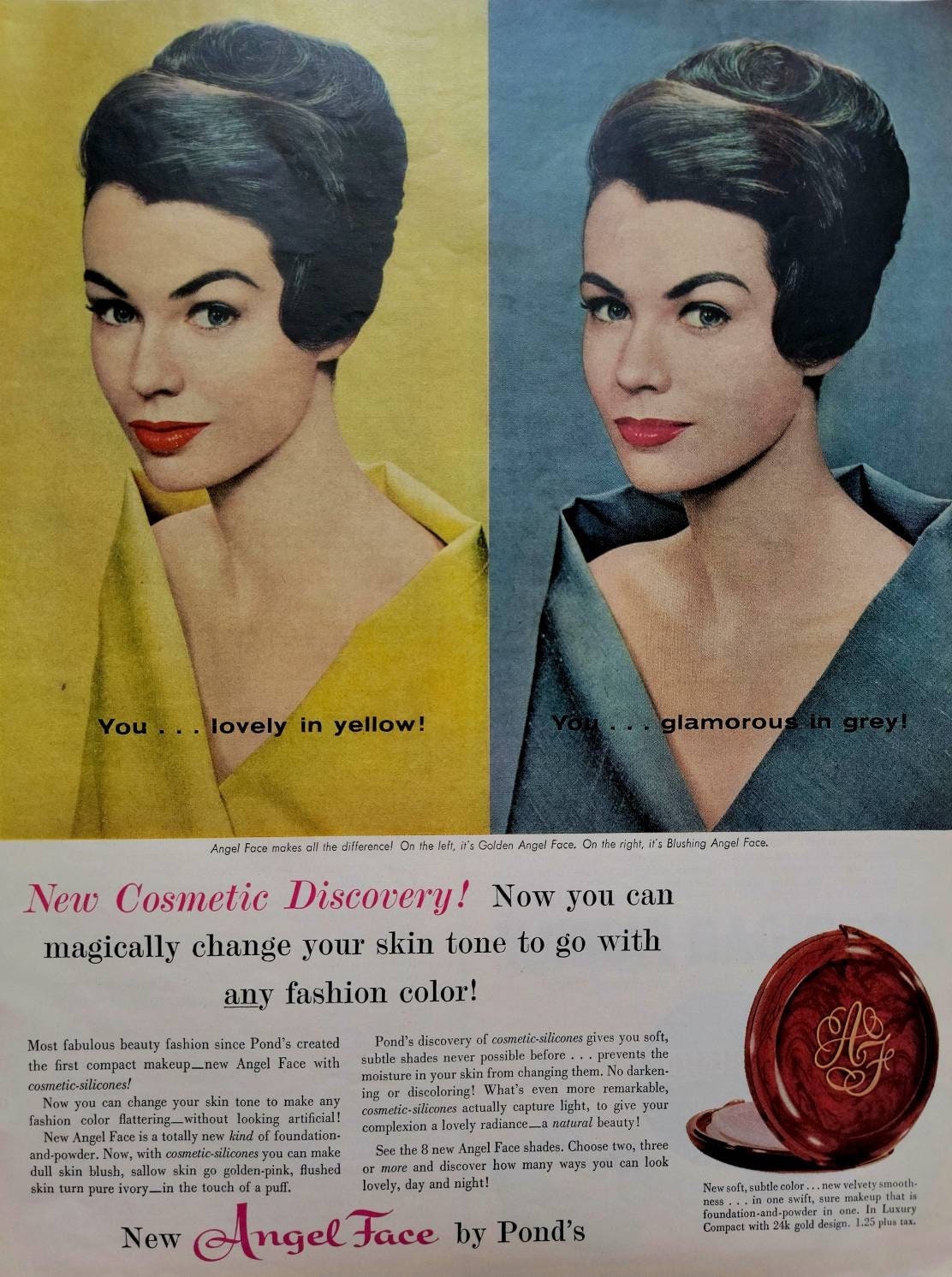This advertisement for Pond's features a stylish portrayal of a woman in two different color schemes. In the first image on the left, she dons yellow attire against a matching yellow background, with text stating, "You... lovely in yellow." Her hair is coiffed into a neat curl, she has arched black eyebrows, and vibrant pink lips. The second image on the right showcases the same woman in a grayish-blue dress and background, with a cape over her shoulders, accompanied by the text, "You... glamorous in gray." Both images highlight her brown, curled hair, neatly trimmed eyebrows, and striking red lipstick.

Beneath these images, in pink, italicized font, the ad declares "New cosmetic discovery." Following in black font, it reads, "Now you can magically change your skin tone to go with any fashion color." Below this, two columns of descriptive text further elaborate on this innovation. At the very bottom, in large text, it promotes "New Angel Face by Pond's." To the right is an image of a glossy, burgundy-red compact with a decorative design, emphasizing the elegance and sophistication of this new cosmetic product.